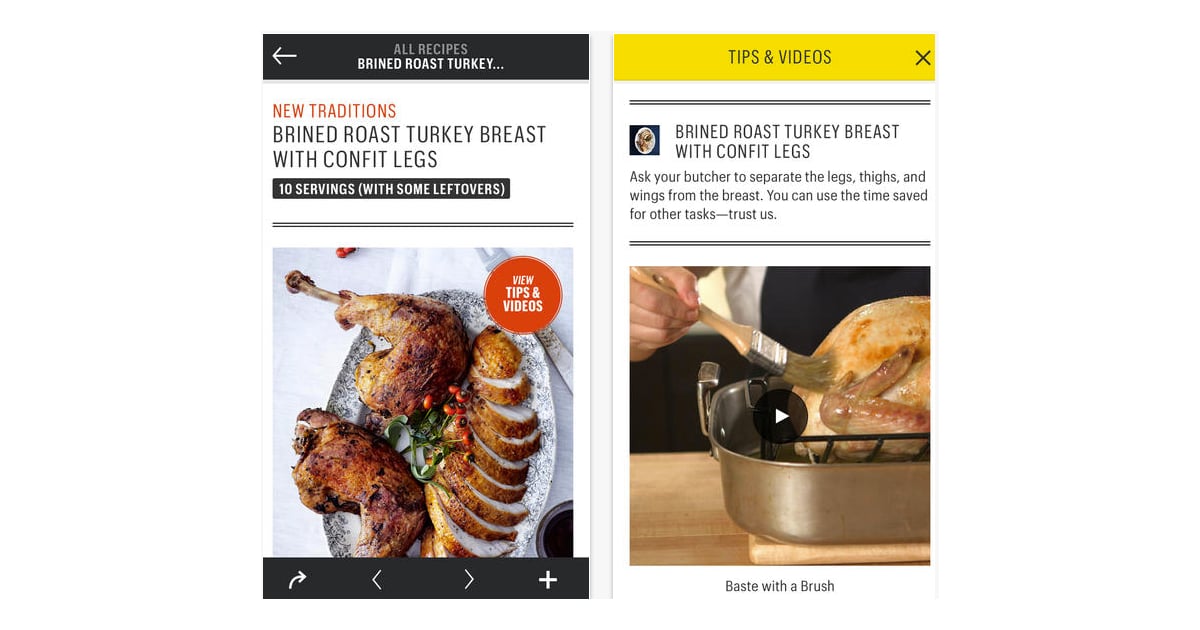The image depicts two side-by-side pages, likely on a mobile device. The left page features the title area in black with a white left-pointing arrow, labeled "ALL RECIPES OF BRINE ROAST TURKEY." Below this, in bold orange text, it reads "NEW TRADITIONS," followed by "BRINE ROAST TURKEY BREAST WITH CONFIT LEGS" in uppercase black letters. A smaller black bar underneath mentions "10 SERVINGS (WITH SOME LEFTOVERS)." 

Below the text is an appetizing image of the meal, showcasing portions of the turkey, including a leg and thigh, neatly arranged on a dish. The dish is accompanied by a small garnishing, possibly a sprig of herbs, and is set on a white table or placemat. An orange circular button reading "VIEW TIPS AND VIDEOS" is also visible on this page.

On the right page, a yellow header states "TIPS AND VIDEOS." The main text reads "Brine a roast turkey breast with confit legs," with additional instructions in lowercase indicating, "Ask your butcher to separate the legs, thighs, and wings from the breast. You can use the time saved for other tasks. Trust us." 

Below this, a video is displayed, showing a turkey being brushed with a marinade or glaze while sitting in a metal pan on a wooden tabletop. The video has the caption "BASTE WITH A BRUSH."